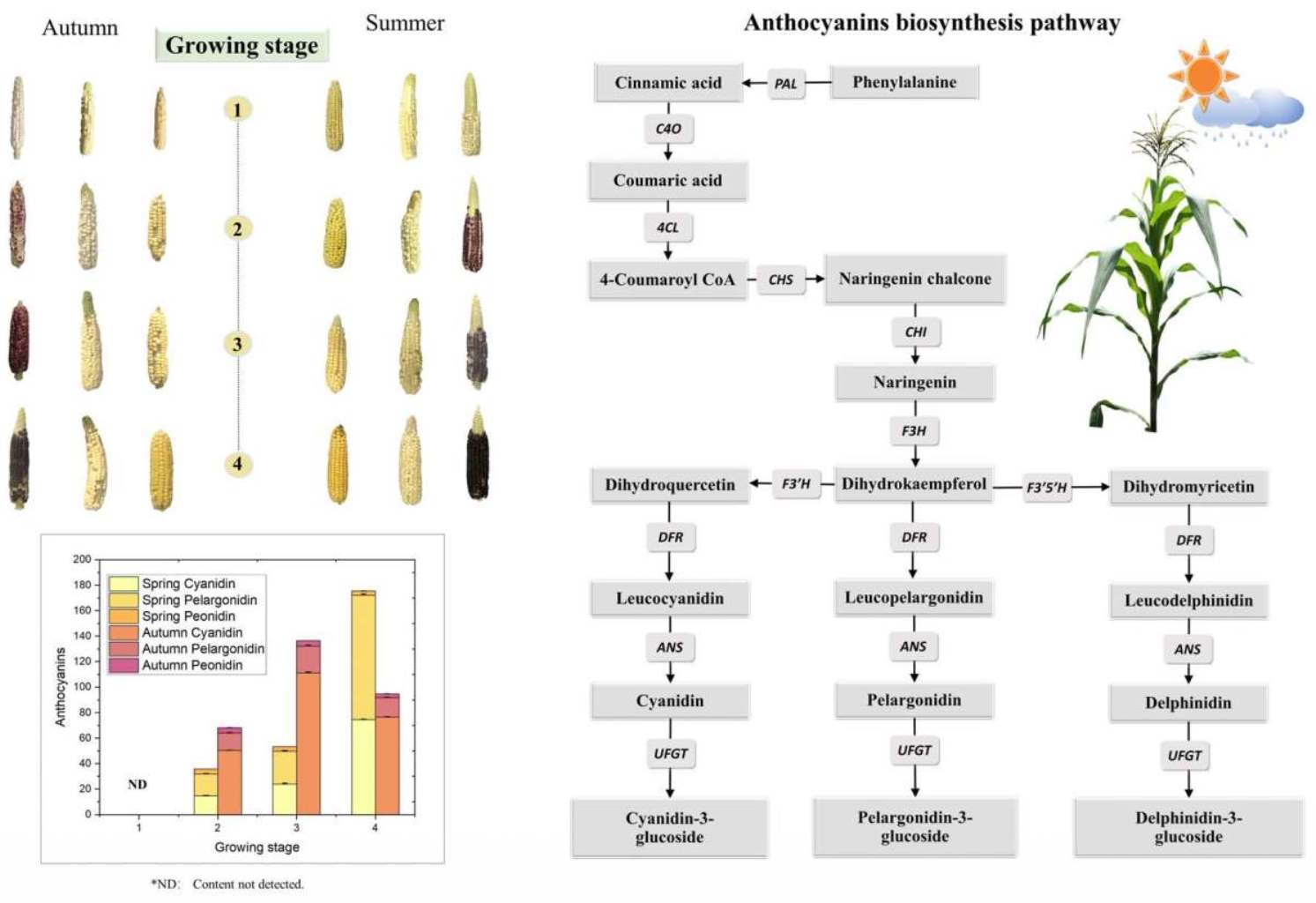This detailed infographic illustrates various aspects of corn growth and anthocyanins biosynthesis. On the top right, the title "Anthocyanins Biosynthesis Pathway" is prominently displayed in black text. Beneath the title, a color illustration of a corn stalk is depicted, flanked by an orange sun and a blue cloud. 

On the left side, the infographic features a flowchart with chemical names in gray rectangles connected by black arrows. Adjacent to this are sections labeled "autumn" and "summer," signaling different growth periods. A central column numbered 1 through 4, in beige circles, displays corresponding stages of corn development, each surrounded by images of the plant at various stages.

Below this section is a bar chart labeled "Growing Stage," with a key in yellow, orange, and reddish hues. The chart correlates the growth stages with anthocyanin levels, providing a visual representation of the biochemical changes in the plant over time.

Overall, the infographic employs a combination of color illustrations, text, and graphic design elements to convey comprehensive information about the growth stages of corn and the associated biochemical pathways.